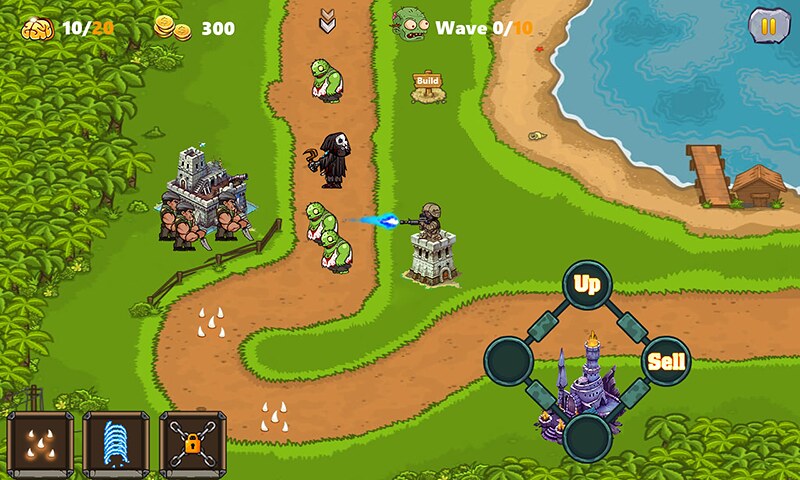This screenshot from an old video game features a brown path that starts on the right, extends straight, makes a large curve, and heads upwards. Along the curve, a wooden fence is placed on one side. To the left of the path, there is a small gray stone castle guarded by three muscular men armed with knives. In the bottom right corner, a mini-map displays a purple castle in the center, encircled by a gray symbol. Additional UI elements include a top round icon labeled "Up" and another on the side labeled "Sail," with two other round icons currently empty. The right side of the scene reveals a large lake with a wooden dock and a small house nearby. A ground sign near the dock reads "Build."